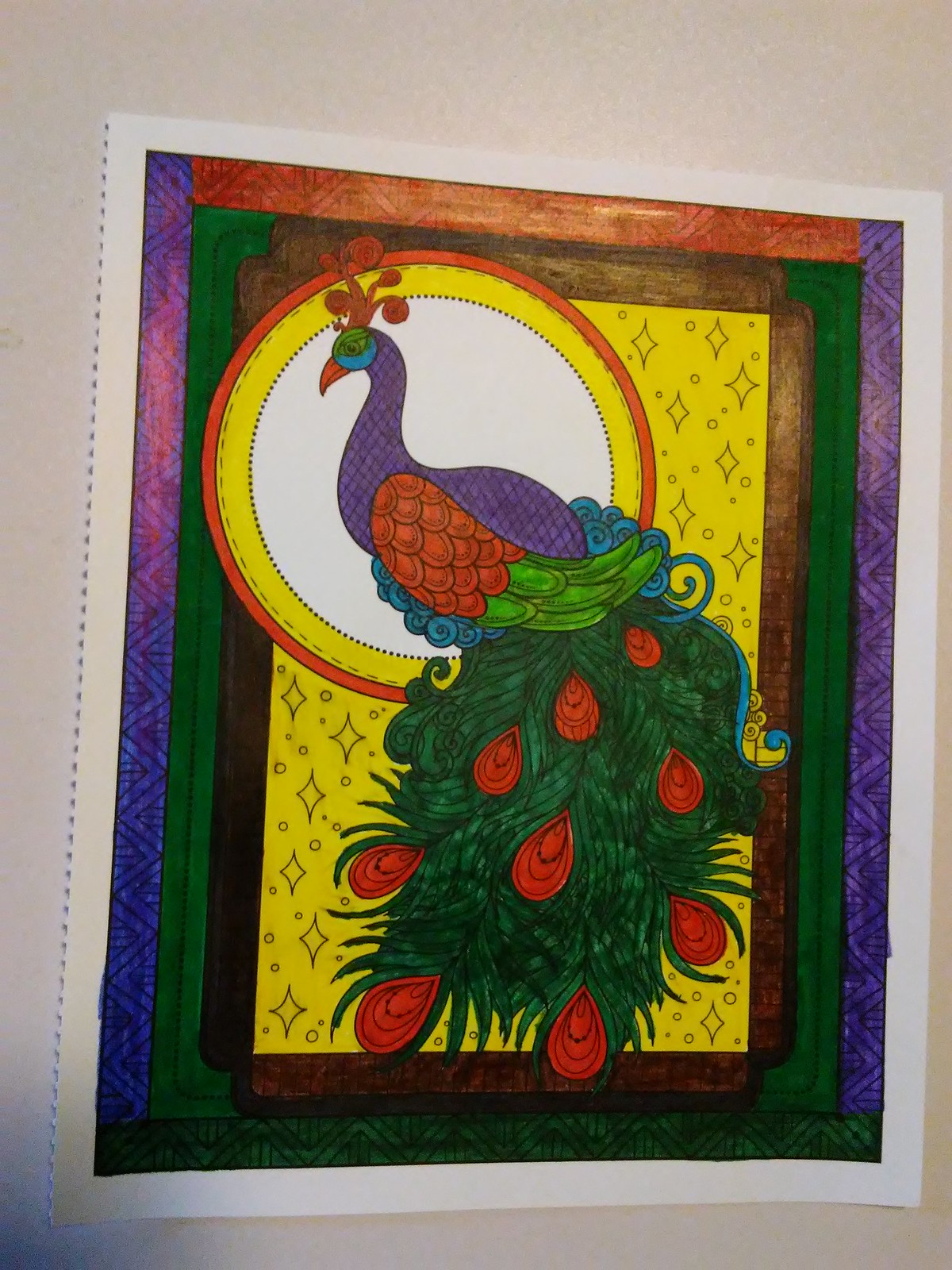This detailed illustration appears to be a fully colored page from a coloring book, torn from a spiral-bound book, and it is placed on a countertop. The image features a vibrant depiction of a peacock, facing left. Its body and neck are predominantly purple, with red head feathers, a blue area around a green eye, and a red beak. The peacock's wing is divided into a scalloped red upper section and a bright green lower section. Flowing down from the bird are numerous dark green, cascading feathers adorned with red teardrop designs, resembling the traditional eye spots found on peacock feathers. 

At the center of the illustration is a white circle, akin to a moon, encircled by a solid yellow line, then a thinner red line, and finally a yellowish-orange border with sparkles. The entire scene is framed by borders in shades of brown, green, orange, and purple. The background of the image is yellow, decorated with small black-outlined diamonds and sparkly shapes, adding an extra touch of whimsy to the vibrant color palette.